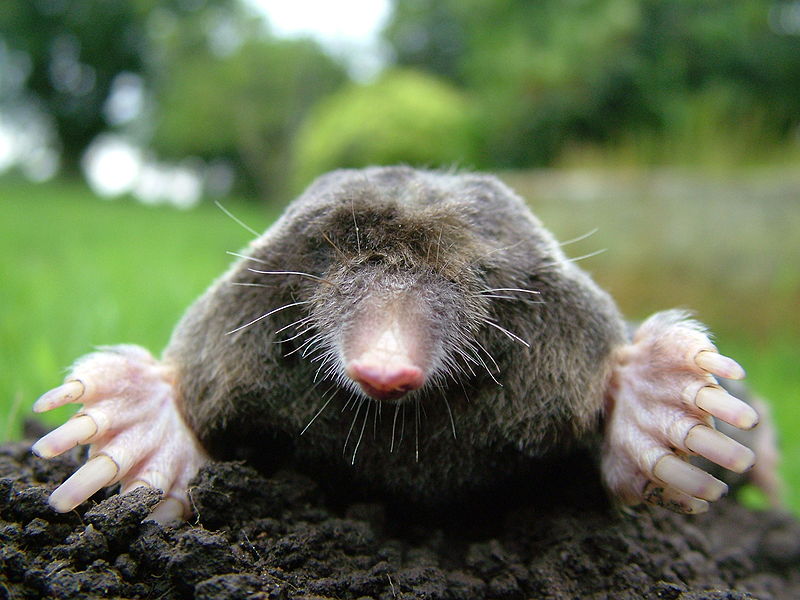This face-on photograph captures a mole above ground, an uncommon sight for these subterranean dwellers known for their poor eyesight. The mole, with its short brown fur, features a notably large and flared pink nose surrounded by an array of whiskers, likely used for sensing its environment. Its front paws, which are prominently displayed, exhibit five long, powerful claws designed for digging through soil. The mole is perched on a clump of brown dirt, possibly pushed up during its burrowing or arranged for the photograph. The background, which is out of focus, reveals greenery with hints of a field and trees bathed in daylight. The image focuses sharply on the mole, emphasizing its details while highlighting the contrast between its natural habitat underground and the unfamiliar surface world.